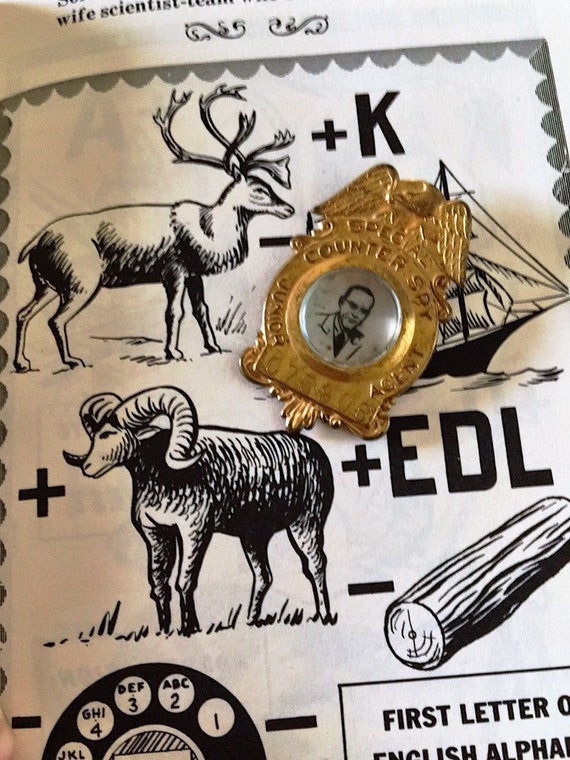The photograph features a brass or gold pin placed on a black-and-white illustrated puzzle sheet. The pin showcases a portrait of a man wearing a white coat and tie, set against a gray or whitish background. Above the portrait, there is an intricately engraved crest resembling bird's wings, and below it, the inscription "Counter Spy" is clearly visible. 

The underlying paper is richly illustrated with various black sketches, including a stag, a goat, a log, a dial phone, and letters such as K, E, D, and L. Additionally, there's an inset located at the bottom right corner indicating "first letter of the English alphabet." The puzzle elements follow a sequence that includes plus and minus signs, suggesting it's a complex word or logic puzzle, possibly a Remus puzzle. 

The pin, with its detailed engraving and historical aesthetic, contrasts sharply yet intriguingly against the monochrome and whimsical illustrations of the puzzle page.